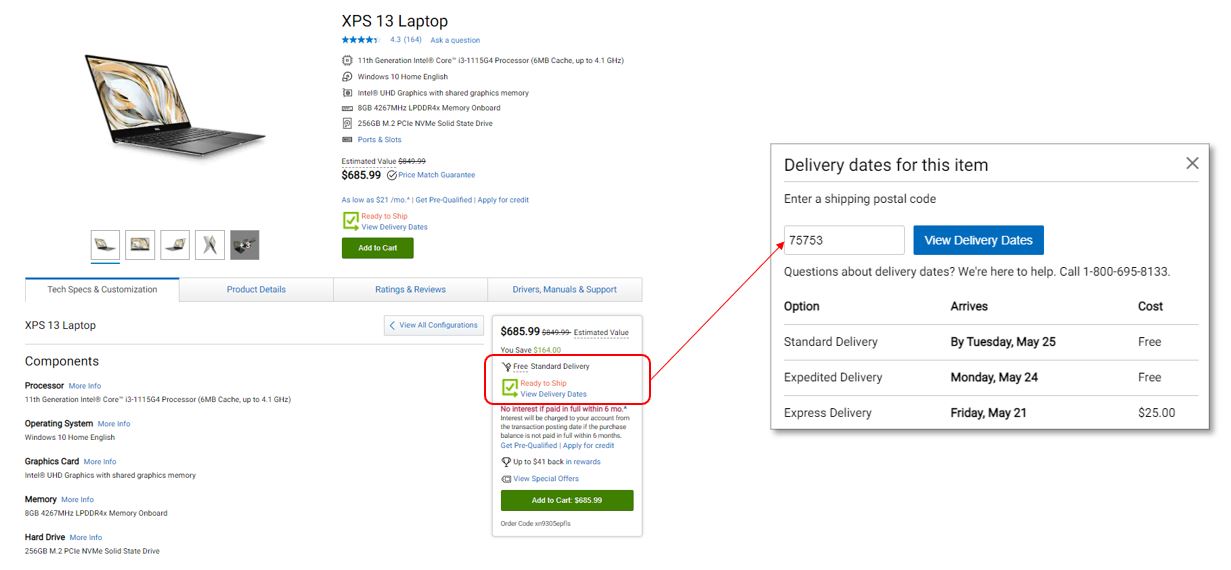This web page highlights the sale of a Dell XPS 13 laptop, featuring a sleek black design complemented by a matching keyboard. The laptop is priced at $685.99 and boasts an average rating of four out of five stars. Prominently, there is an 'Add to Cart' button for easy purchasing.

The website includes navigational tabs for "Tech Specs and Customization," "Product Details," "Ratings and Reviews," and "Drivers, Manuals, and Support." Key specifications include an 8 GB memory, a 256 GB hard drive, and Windows 10 Home Edition as the operating system. Some details regarding the processor and graphics card are not fully visible.

A special notice, highlighted in red with an arrow pointing to a section on delivery dates, captures attention. Shoppers are prompted to enter a shipping postal code (example given: 75753) and can click the blue "View Delivery Dates" button for more information. There’s also a "Questions about delivery dates?" section with a help number: 1-800-695-8133.

Delivery options outlined include:
- Standard Delivery: Arrives by Tuesday, May 25th, free of charge.
- Expedited Delivery: Arrives by Monday, May 24th, free of charge.
- Express Delivery: Arrives by Friday, May 21st, for an additional $25.